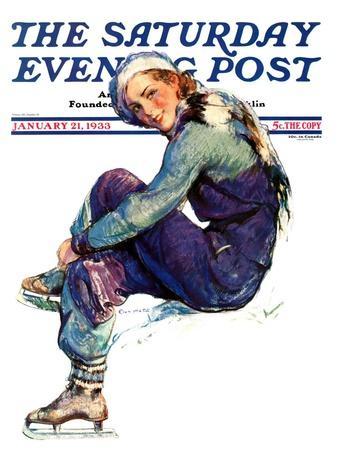The image showcases the cover of "The Saturday Evening Post" from January 21st, 1933, priced at five cents per copy. The top of the cover features the magazine's title in blue against a white background, with obscured text behind the main illustration. The cover art depicts a smiling woman with curly red hair, sitting and putting on ice skates. She is adorned in a coordinated outfit, consisting of a light green and dark purple sweater and pants, a white and brown scarf, and a white and blue cap. Her ice skates feature brown shoes with silver or white blades. To the left of the woman, the date "January 21st, 1933" is displayed, while "Five Cents the Copy" is noted to the right. There are additional lines of red and blue text both above and below her image, suggesting further information about the magazine.